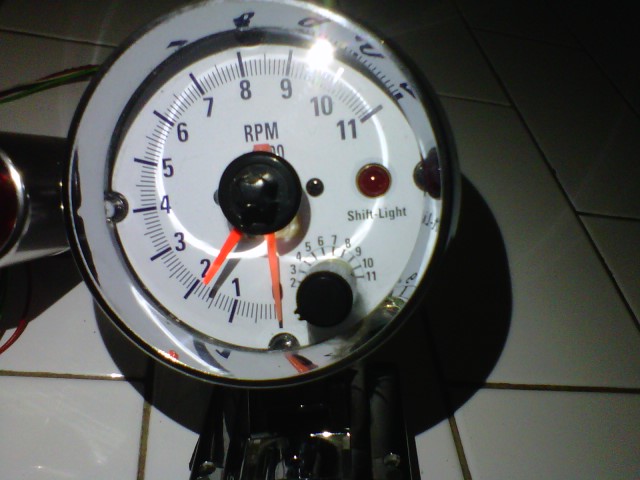This detailed close-up photograph showcases a tachometer, likely from an automobile. At the center of the device, the letters "RPM" are prominently displayed, indicating it's used to measure revolutions per minute. The face of the tachometer features large black numerals ranging from 0 at the six o'clock position, sweeping counterclockwise up to 11 at the two o'clock position. Between each numeral, several smaller black lines incrementally divide the spaces.

Notably, at the three o'clock position, a small red light labeled "Shift Light" sits just below the numeral 11, currently unlit. Beneath this, a dial with numbers 2 through 11 occupies the upper semicircle, used presumably to set the shift light threshold. The instrument’s vibrant orange hands contrast sharply against its background for easy readability.

Encircling the dial is a gleaming, metallic silver bezel, adding a touch of sophistication. The tachometer rests on a floor with white tiles, casting a shadow behind it in the otherwise dimly lit background. A light source, likely a camera flash, illuminates the instrument, accentuating its details.